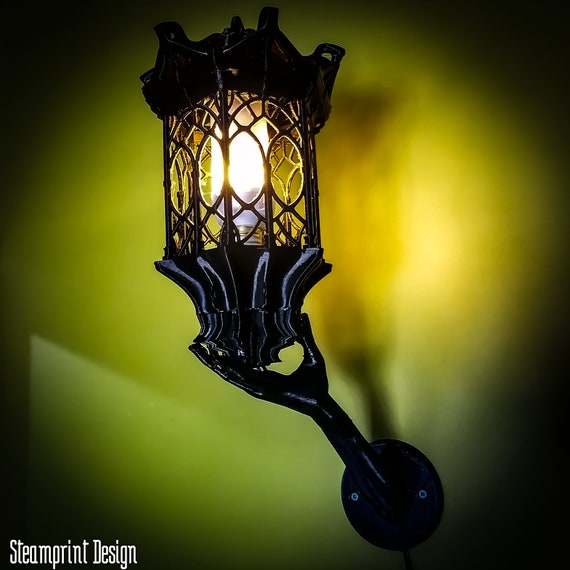This indoor photograph showcases a unique and intricately designed lamp featuring a distinct combination of modern and old-fashioned elements. Central to the image is a black metal arm and hand, seemingly realistic and detailed, extending from a circular, metal base that is securely screwed into a wall. The sophisticated hand design, with its thumb and fingers carefully gripping an intricate, jagged lantern casing, is particularly striking. The lantern itself is capped with black metal on both the top and bottom, encasing a specially designed light bulb that emanates a bright, distinguishable glow, unlike that of a traditional candle. The wall behind the lamp is a lime green or yellow color, adding a contrasting backdrop that accentuates the lamp's features. In the lower left of the image, the words "steam print design" are written in white text, indicating a possible stylistic or brand element. Overall, the ornate lamp appears to fuse historical aesthetics with contemporary technology, making it a captivating focal point in the room.